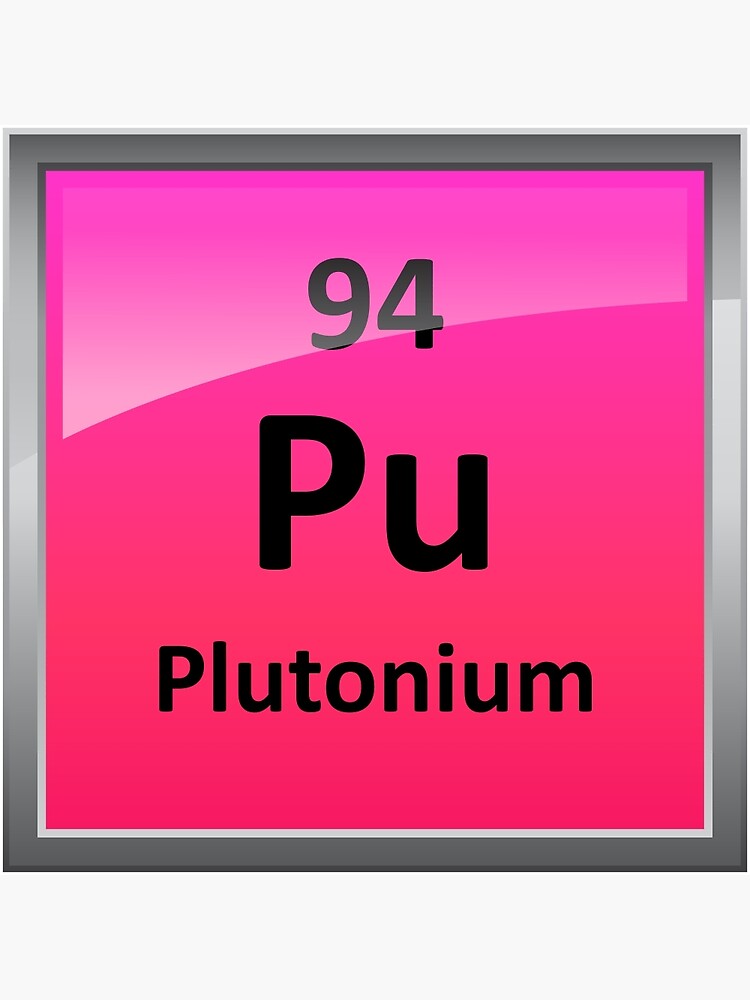The image showcases a close-up of the periodic table entry for plutonium, prominently featuring the atomic number 94 and the symbol Pu in large black text. Below this, in smaller black text, is the name "plutonium." The background of the cell transitions from a pinkish purple to a bluish purple gradient, set within a sleek silver frame that appears to be behind glass. There's a noticeable sheen or reflection at the top part of the image, particularly over the number 94, although it's unclear whether this is part of the design or a photographic artifact. The bright and vivid colors of the background provide a striking contrast to the black text, making the plutonium entry a visually captivating piece of art. White edges of the background are visible around the framed section, enhancing its framed, artistic presentation.